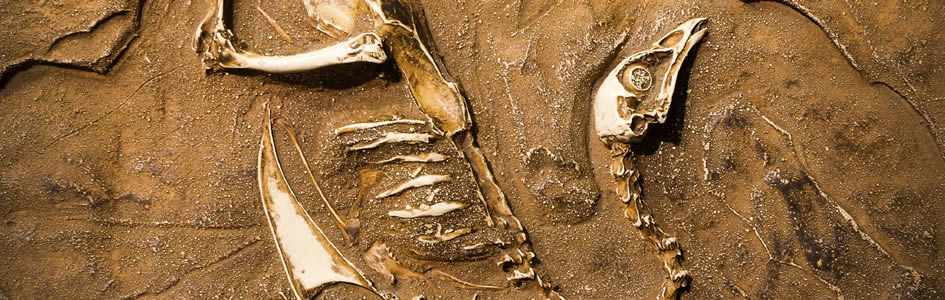The photograph depicts an archaeological dig revealing the partially unearthed fossilized remains of a bird-like creature embedded in a brownish, sandy soil. Dominating the image is the excavation site, where meticulous digging has exposed significant portions of the skeleton. A notable neck stretches out, culminating in a head characterized by a pronounced beak and visible eye socket. Although the full body isn't visible, one can see the ribs extending from the vertebrae, and a robust back leg with an extended foot. Additionally, there appears to be a wing structure and something resembling a dorsal fin beneath the area that would correspond to the belly. This intricate scene captures the ongoing process of uncovering the ancient bones, blending the meticulous art of archaeology with the mystery of paleontological discovery.